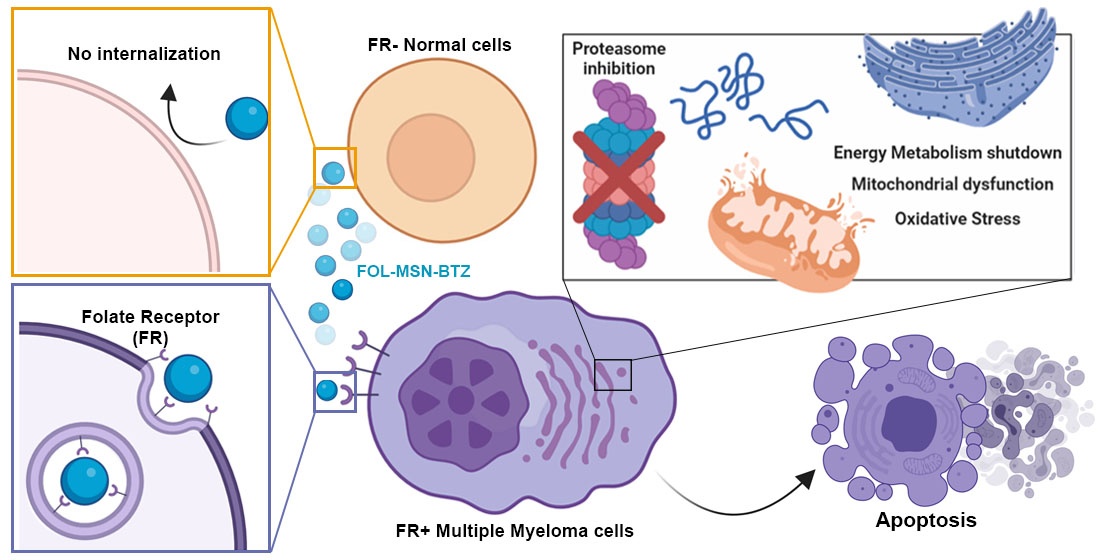The image is a detailed, color-coded medical illustration depicting the interaction and breakdown of different cell types. 

On the top left, there is a yellow box labeled "no internalization" featuring a pink half-circle next to a blue sphere with an arrow pointing away from it. Below that, a purple box is labeled "folate receptor (FR)" and shows a blue sphere successfully entering a half-circle, indicating how folate receptors work. 

To the right of these boxes, more detailed explanations are provided. At the top, an orange circle, labeled "FR normal cells," shows a dark orange nucleus and has blue spheres around it labeled "FOL-MSN-BTZ." Below, a purple, irregularly shaped blob, labeled "FR plus multiple myeloma cells," displays a complex, cellular structure with indentations and purple-orange segmented shapes.

On the right side of the image, a black-framed box contains several smaller illustrations. One picture, labeled "proteasome inhibition," shows a pile of purple, blue, and pink spheres crossed out with a red X. Another, an orange bean-shaped object, is labeled "energy metabolism shutdown, mitochondrial dysfunction, and oxidative stress," featuring blue squiggles and other shapes emphasizing cellular stress processes.

At the bottom right, another purple blob with light purple lobes and a darker purple center is labeled "apoptosis," illustrating the cell disintegration process. 

Overall, the diagram visually explains how cells, particularly cancer cells like multiple myeloma, interact with various treatments and undergo processes leading to their breakdown and death.